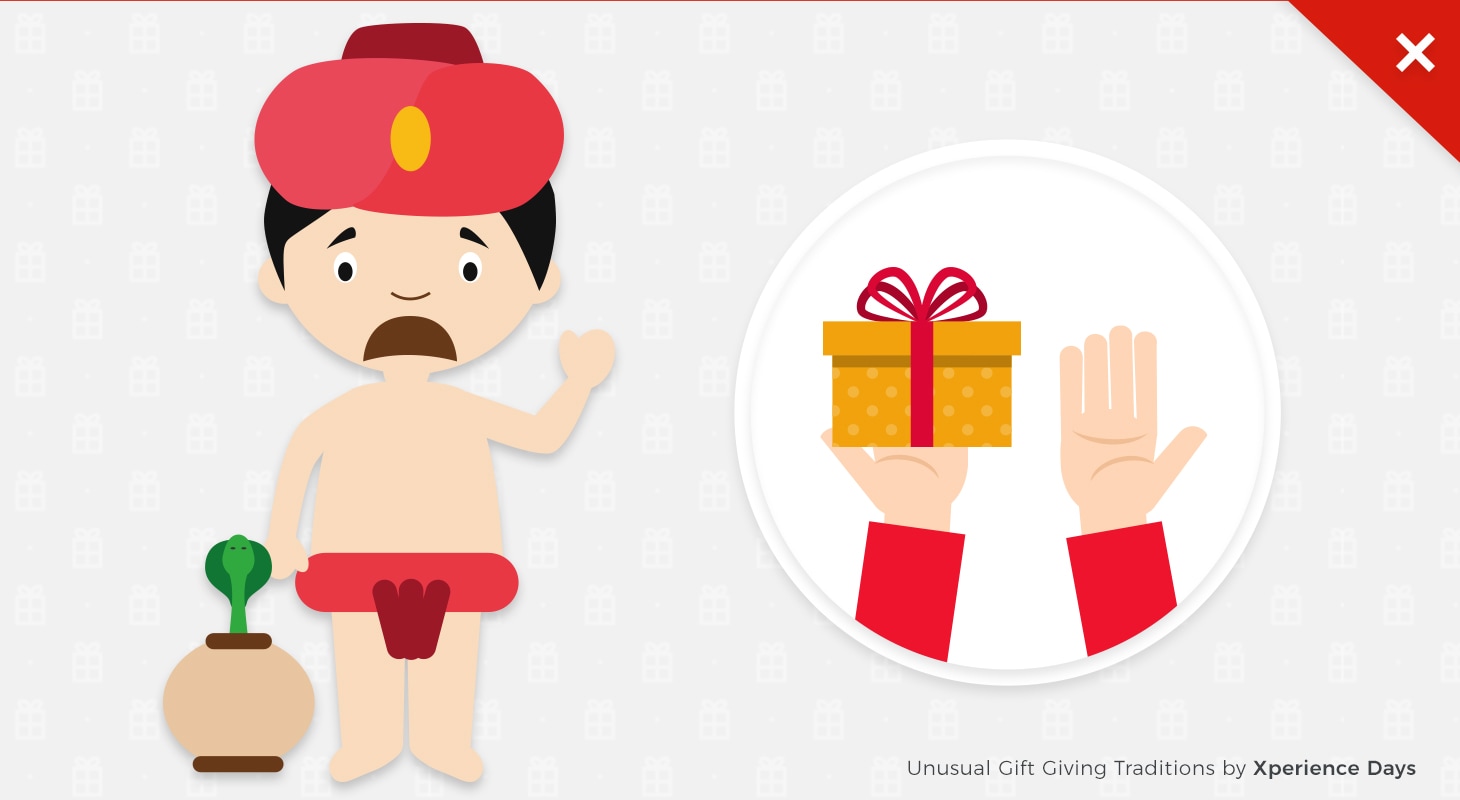The illustration, titled "Unusual Gift-Giving Traditions by Experience Days," depicts a cartoon snake charmer, who is a small boy with white skin, very dark black hair, and a downturned mouth in a look of displeasure. He wears a red turban with a yellow gem and a red loincloth. Positioned next to him is a brown urn with a green cobra peeking its hooded head out. In a white circle to the right, there are two hands with red sleeves; one hand is empty, while the other holds a gold-wrapped gift box with a red ribbon. In the upper right corner, there is a red "X" sign.